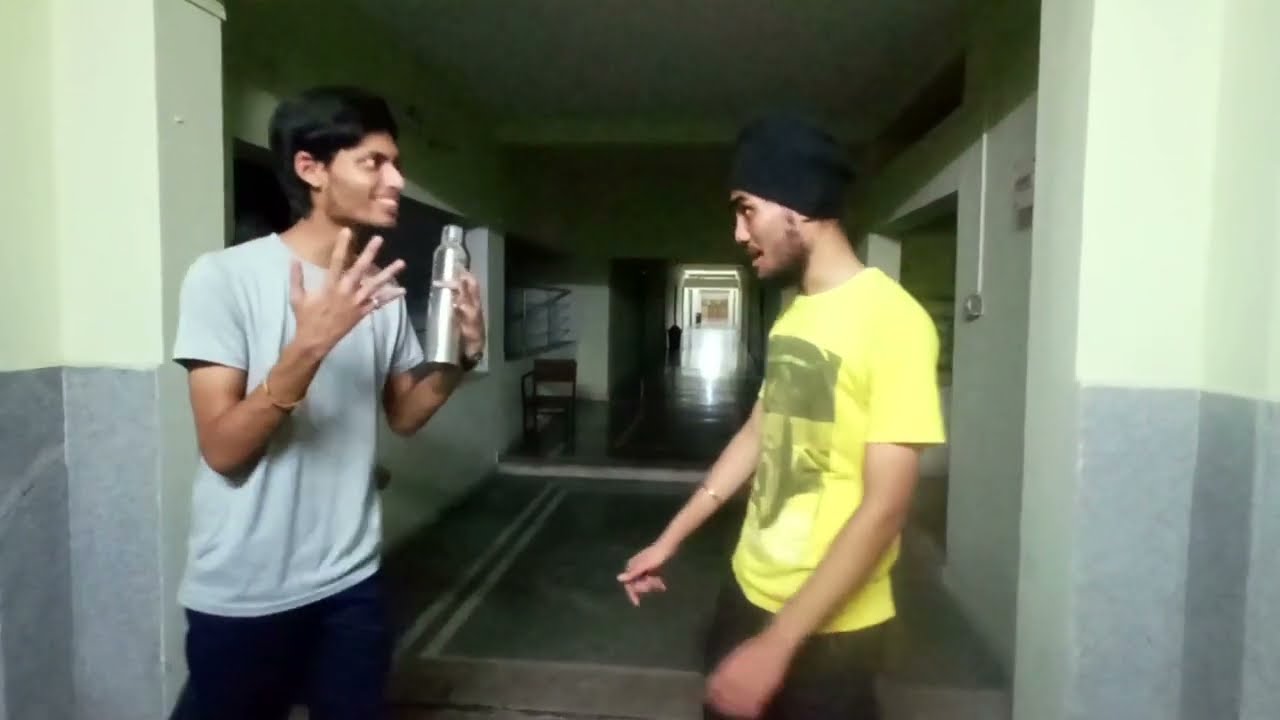The image depicts two young men, who appear to be of Indian or Middle Eastern descent, engaging in a conversation in a dimly lit hallway of a public or apartment building. The hallway extends into a long, dark corridor with light at the end. Behind the men, there's a rug and a chair, adding depth to the scene.

On the right stands a man in a yellow t-shirt with an indiscernible design, paired with dark shorts. He has a short beard and wears a dark hat or beanie, his arms relaxed by his sides. Opposite him, the man on the left has short black hair and wears a gray or light blue t-shirt with dark pants. He holds a silver thermos or water bottle in his left hand and raises his right hand, gesturing animatedly as if explaining something. The intensity of the discussion is evident in their expressions and body language.